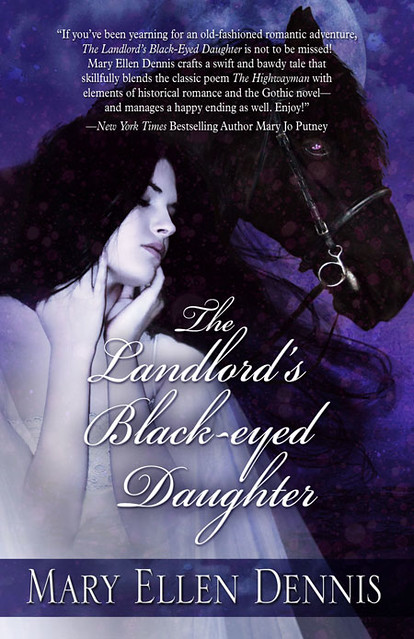This image is the cover of a novel entitled "The Landlord's Black-Eyed Daughter" by Mary Ellen Dennis. The cover features a tall, rectangular shape with a predominantly purple background that resembles a night sky, complete with lighter shades and faint clouds. On the left, there is an image of a woman with alabaster skin and long black hair. Her hands are raised to her neck and cheeks, and her face is tilted downwards to the right, her eyes almost closed, giving her a pensive expression. She is wearing a white gown. Standing behind her to the right is a dark reddish-brown horse with spots on its face, its head positioned at the top right corner of the cover. The title of the book is written in elegant white cursive font across the woman’s chest and shoulders, and below it, in white capital letters over a purple rectangle, is the author’s name, Mary Ellen Dennis. At the top, a six-line paragraph from New York Times best-selling author Mary Jo Putney praises the novel, describing it as an old-fashioned romantic adventure. The overall color scheme consists of purples, blacks, blues, dark browns, and whites.